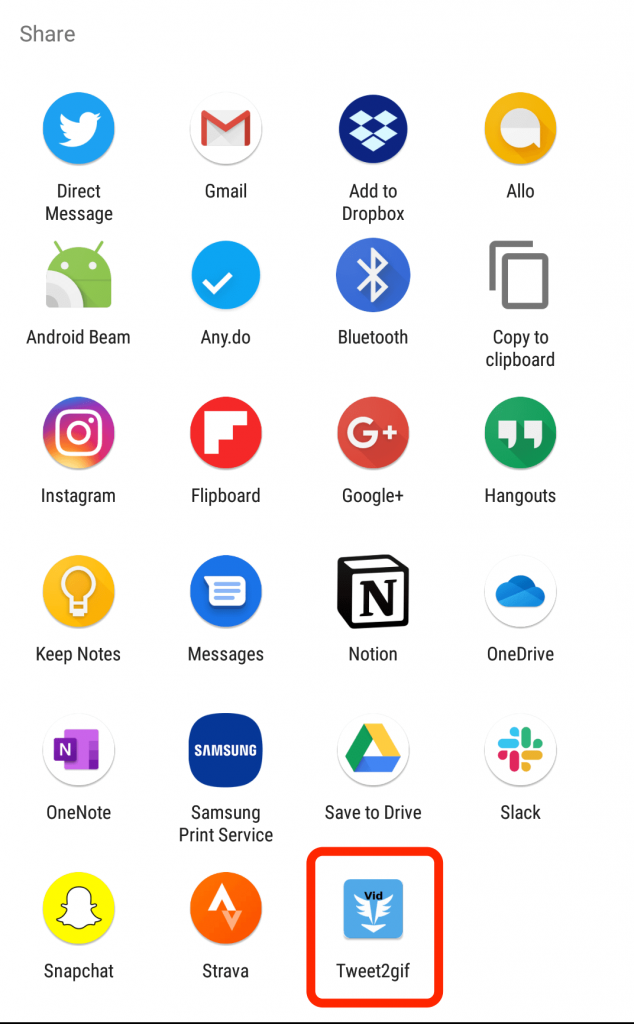The image displayed is a screenshot of a smartphone's app-sharing screen. At the very top, in a straightforward black and white design, the word "Share" is prominently written. Directly beneath, a collection of various app icons is neatly arranged. Starting from the top row, the apps include Twitter, Direct Message, Gmail, Add to Dropbox, and Allo. 

The next row features Android Beam, Any.do, Bluetooth, and Copy to Clipboard. Following this, additional app icons are visible for Instagram, Flipboard, Google+, Hangouts, Keep Notes, Messages, Notion, OneDrive, and OneNote. Continuing down the list, Samsung Print Service, Save to Drive, Slack, Snapchat, Strava, and Tweet to GIF are also present. Noteworthily, the icon for Tweet to GIF is distinctly highlighted with a red box, drawing special attention to it. This comprehensive screenshot effectively captures the wide array of app-sharing options available on the device.